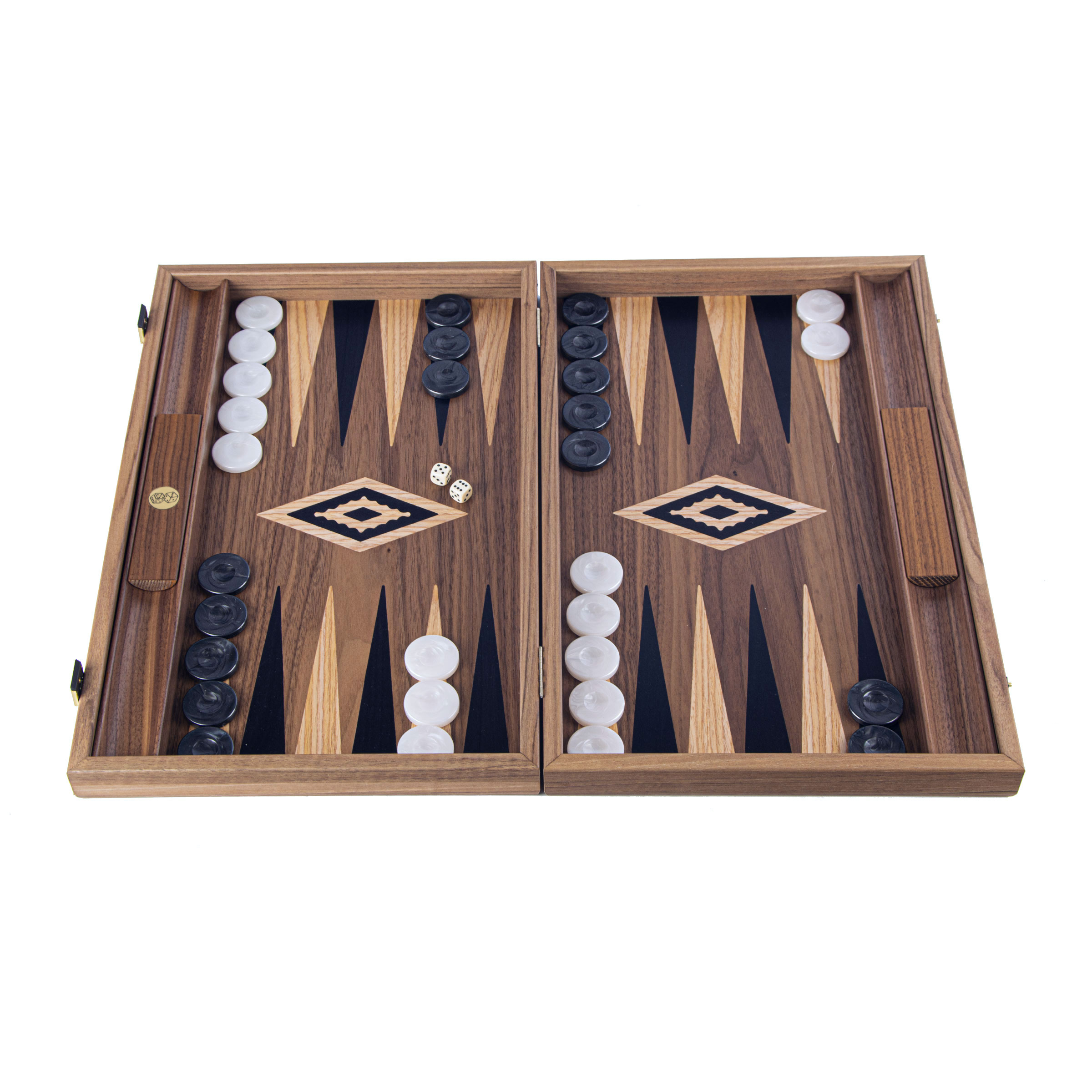The image portrays a high-quality, old-fashioned backgammon set, beautifully crafted from dark wood and designed like a suitcase-style hinged box that opens flat to reveal the game board. The backgammon board features intricate inlays, with alternating dark black and light brown wooden triangles that create a visually striking pattern. The central focus of the image is on the board, which is ready for play, displaying a set of white and black round, disc-like game pieces—seven of each color neatly arranged. Additionally, two dice are positioned on the left-hand side of the board showing a roll of 6 and 5, indicating the game is set for action. The detailed craftsmanship and classic design emphasize its vintage appeal and readiness for play.